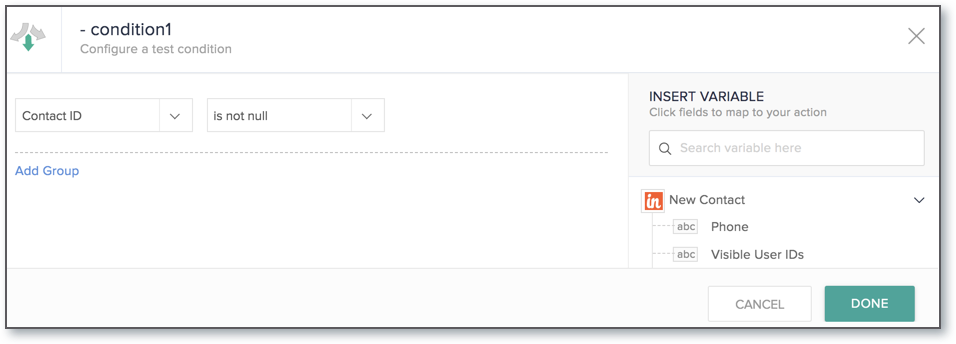In the image, the top-left corner features a label that reads "Condition 1, Config and Test Condition" in black text against a white background. Adjacent to this text is an icon depicting three arrows: one pointing left, one pointing right, and one pointing downward. The downward-pointing arrow is colored green, while the other two arrows are grey. Below this icon is the text "Contact ID" next to a drop-down menu, which shows "Contact ID" as the selected option. To its right is another drop-down menu with "Is Not None" selected. 

Below these elements, "Add Group" is written in blue. On the right side of the image, there is a section titled "Instance Variable" with accompanying instructions that read "Click Fields to map your action." Underneath this section is a search box labeled "Search Variable here." Additionally, the text reads "New Contact. Phone, Variable, Visible User ID." 

To the left of "Contact," there is a small, red, square icon with the text "In" written in white. In the bottom-right part of the image, there are two buttons: "Cancel" on the left, which is white, and "Done" on the right, which is green with white text. The overall page features a detailed border with a black outline and has a black box around the home page section.